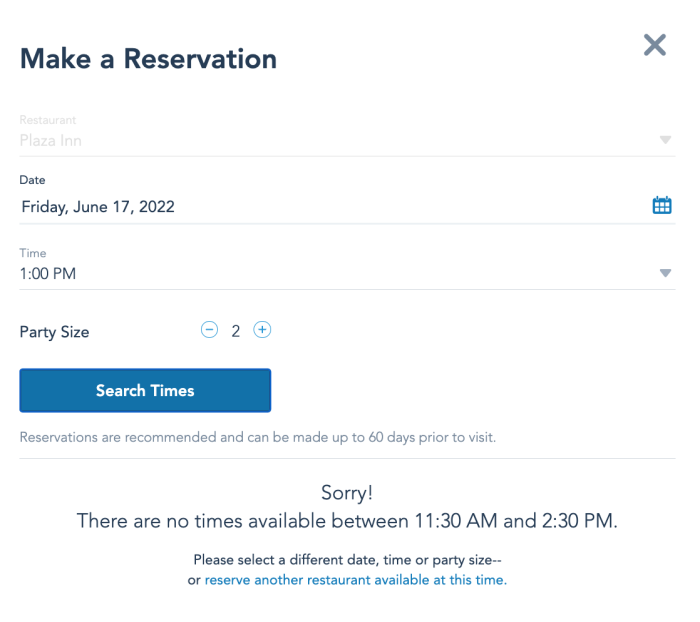**Screenshot of a Reservation Attempt on an Unspecified Website**

In the upper left-hand corner of the image, the title "Make a Reservation" is prominently displayed in the largest font. The upper right-hand corner features a small "X" icon for exiting the webpage. The overall background is predominantly white.

On the left side of the image, there are three main search bars. The first allows for the selection of the restaurant. The second search bar is set for the date "June 17th, Friday, 2022." The third search bar indicates the desired time of "1 p.m." Below these, there is an option for selecting the party size, with plus and minus buttons in blue to adjust the number of people.

At the very bottom of the page, a message indicates that no available times can be found between 11 a.m. and 2:30 p.m. It reads: "Sorry, there are no times available between 11 a.m. and 2:30 p.m. Please select a different date, time, or party size, or..." Following this, a clickable blue link suggests users "Reserve another restaurant available at this time."

This image clearly captures the unsuccessful attempt to make a reservation, highlighting the need for alternative options due to the unavailability of the desired time slot.